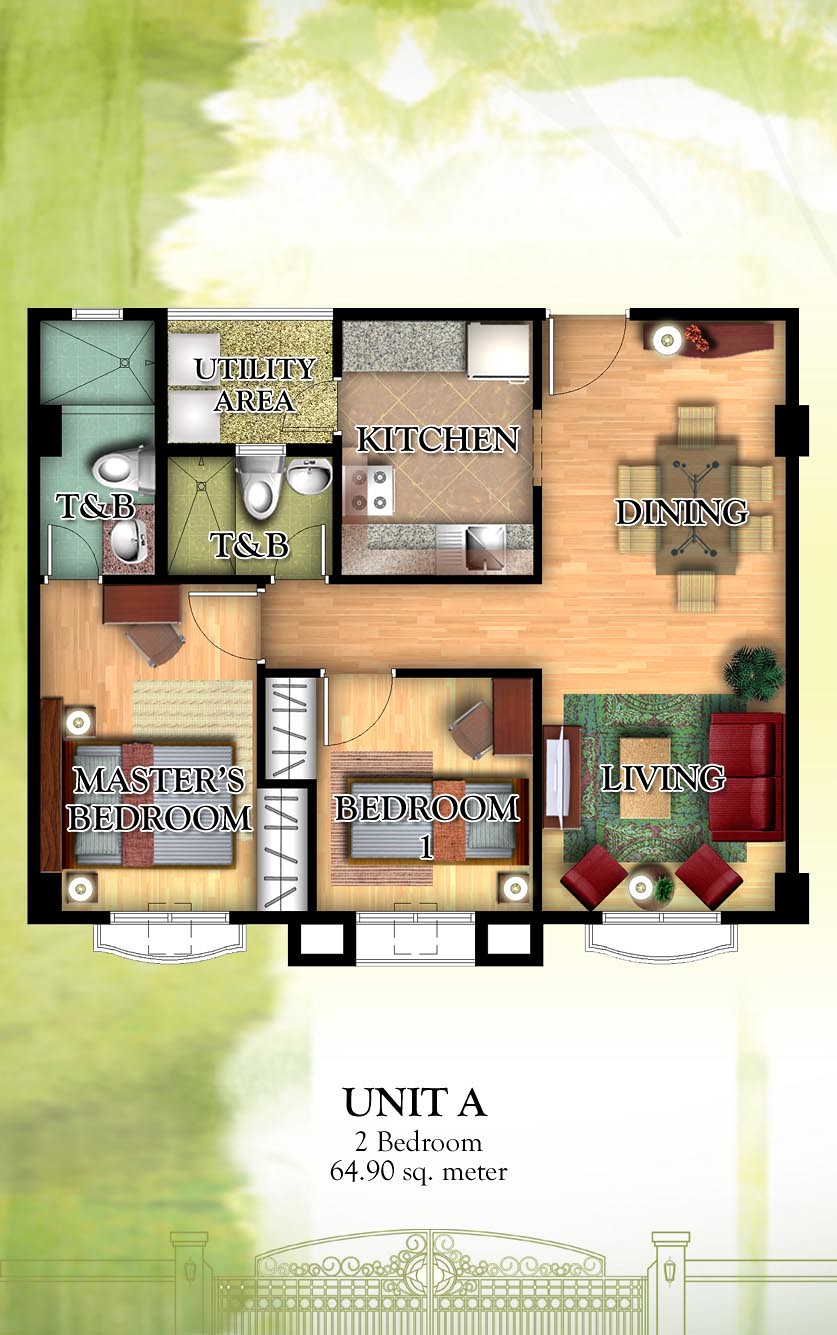This is an illustrated floor plan for an apartment, set against a background featuring a greenish-yellow hue with large white splotches. The floor plan, roughly square in shape, delineates various sections of the residence using blocked-off squares and rectangles. The floor within each section is depicted with a light brown wood grain pattern.

On the left side of the floor plan, there are two separate areas labeled "T and B," each indicating the presence of a toilet and sink. Above these, there is a section labeled "Utility Area." Adjacent to the utility area on the right, the "Kitchen" section shows icons representing a sink and stove. 

Next to the kitchen, an open area labeled "Dining" connects to another open space below it called "Living." This living area includes red and green sections denoting likely positions for a couch and chairs. To the left of the living area, a section marked "Bedroom 1" contains smaller icons representing a cabinet and a bed. Adjacent to Bedroom 1, on the far left, is the "Master's Bedroom," which also includes a bed representation.

The plan also includes markings for windows and features a label in black print identifying the unit as "Unit A," with specifications of "2 bedrooms, 64.90 sq. meter." Beneath the main floor plan, there is a line drawing that illustrates a wrought iron gate flanked by walls on either side.